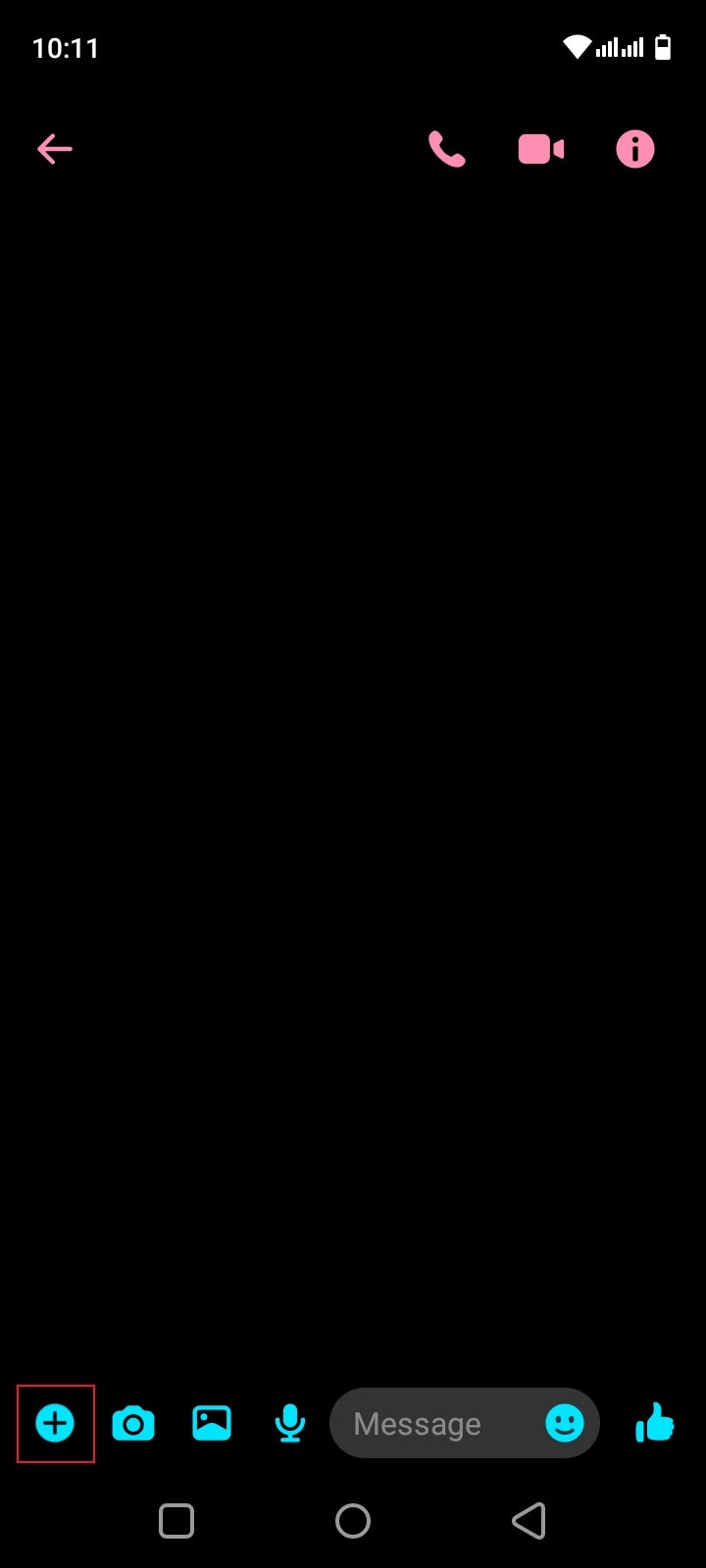The screenshot from a cell phone display was taken at 10:11 AM, as indicated in the upper-left corner of the screen, with a battery level of approximately 50% shown on the upper right. The main background of the screenshot is entirely black, suggesting a possibly failed image capture. The interface featured in this screenshot includes various controls in pink, located at the top portion of the display. On the left side, there is a left-facing arrow, while the right side displays icons for phone, camera, and information.

Dominating the center of the screenshot is the black background, devoid of content. However, the bottom toolbar stands out with a series of interactive buttons. Most prominently, a blue circular button with a plus sign in the center is highlighted with a red square. Adjacent to this are additional icons: a camera, a gallery icon, a microphone, a message box featuring a smiley face, and a thumbs-up symbol. These icons are all rendered in a light blue color, providing a sharp contrast against the dark background.